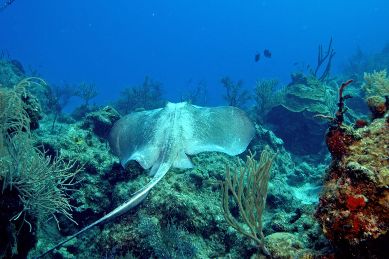The captivating underwater image showcases a stunning coral reef teeming with marine life. Dominating the scene is a graceful stingray, captured from behind as it glides serenely between two prominent coral formations. The stingray's tail, black-tipped and spear-shaped, transitions from black to gray as it meets the lighter gray body, all culminating in darker gray wings. The coral structures are vibrant; one is a striking orange, while the other appears green, adorned with moss. Surrounding the stingray are various types of corals, including leaf coral and bubble coral, along with sea anemones, adding texture to the underwater landscape. To the front of the stingray, about 20 feet ahead, swims a small school of black fish, contributing to the bustling marine activity. The background is a deep, overwhelming blue, highlighting the rich biodiversity and serenity of the underwater world.